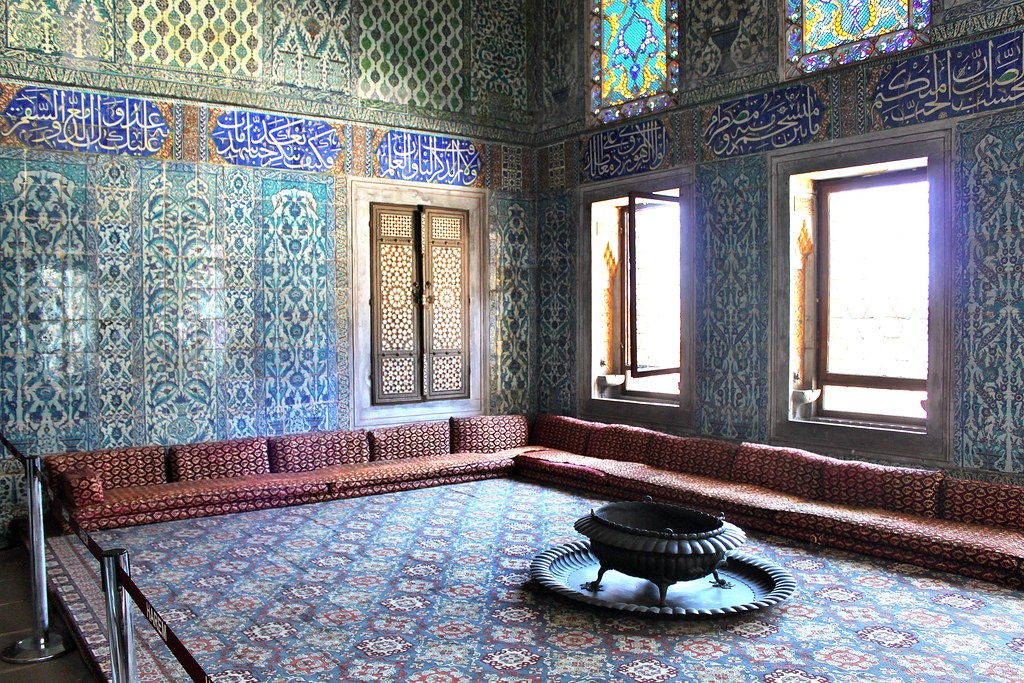The room depicted in the image appears to be a richly decorated interior, possibly of a mosque or a section inspired by Persian design. The room features intricate walls adorned with a blend of turquoise blue, darker blue, green, gray, off-green, tan, and white colors, all contributing to a distinct Persian aesthetic. Additionally, there are elements resembling stained glass or intricately painted panels.

Dominating the center of the room is a black metal fire pit or brazier with four legs, elevated above a metal tray. The fire pit is currently not in use. The flooring is a highly ornate Persian carpet, enhancing the room's traditional vibe.

Running along the left side, curving around the corner, and stretching along the right side, is a low, legless seating arrangement upholstered in a dark brownish-red, ornate fabric. This seating resembles a large sectional couch. Above this seating are two large, open square windows and a partially ajar set of double doors.

Farsi text and non-figurative illustrations adorn some of the walls, reinforcing the cultural and historical ambiance of the room. Silver columns with a velvet rope create an area that guests must stay behind, adding a touch of exclusivity to the space.